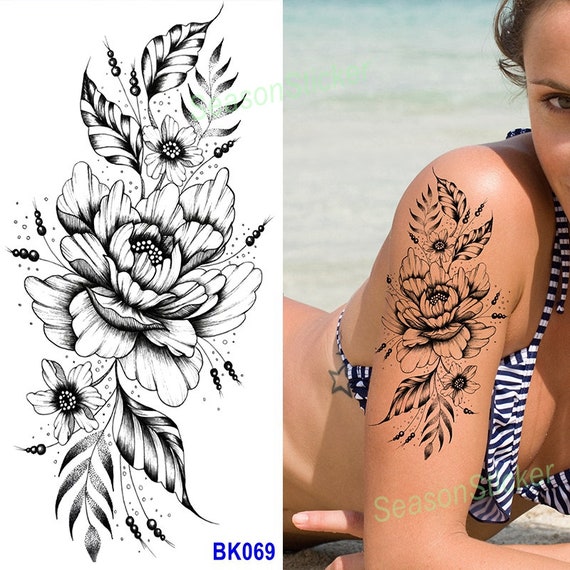The image showcases a detailed and vintage-style black and white floral tattoo design labeled with the product code BK069. The tattoo features intricate line work, stippling, and shadowing, adorned with flowers, leaves, vines, and berries. This design is displayed twice within the image: first as a standalone artwork and second applied onto a woman's left arm, extending from her shoulder to about two-thirds down her upper arm. The woman, a tanned, dark-haired individual with a teasy look in her visible eye, is clad in a tiger-striped or black and white bikini. She's lying on her stomach on a sandy beach with light greenish-blue ocean water in the background. Her hair appears wet and pulled back, suggestive of a recent dip in the water. Additionally, she has a real star tattoo outlined in black ink on her ribcage. The image also includes a watermark at the top and bottom that reads either "Season Seeker" or "Seasoned Soaker," likely indicating the brand or theme for the temporary tattoo.